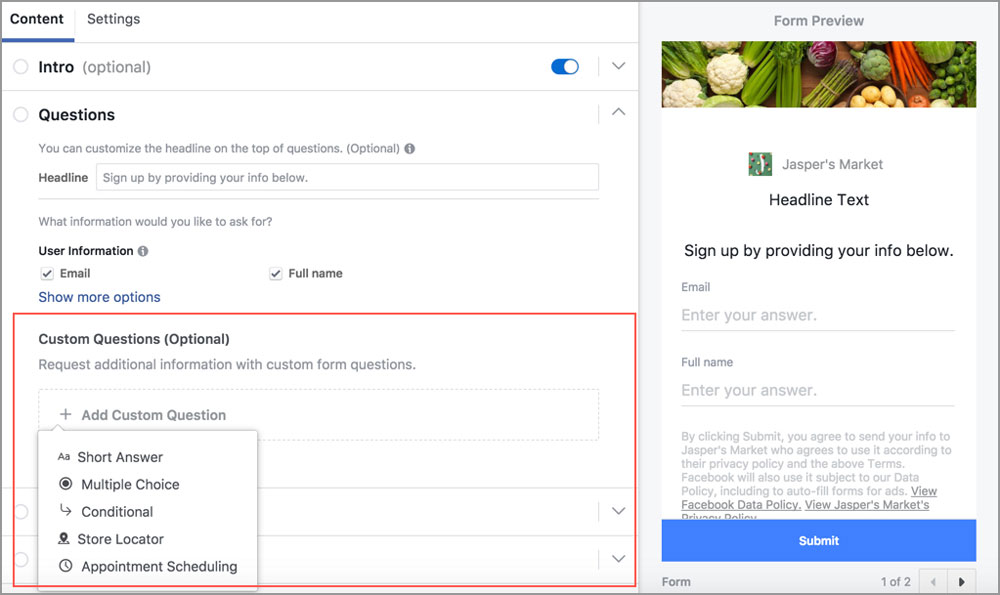The image displays a content management interface for customizing a form. On the left side of the page, there's a navigation pane titled "Content and Settings," specifically focused on the "Content" section. This pane outlines various options or sections of the site. On the right side, there's a preview pane labeled "Form Preview."

Within this preview, a sample form for "Jasper's Market" is displayed. It features placeholder elements including a headline text that reads, "Sign up by providing your info below," alongside fields for email and full name. Below these fields, there's some placeholder legal text followed by a prominent blue submit button.

Back on the left, the user can select different elements of the form to customize, including an introductory text, various question sections, and headline text. Users can specify which text fields they want to include, for example, unchecking the email field if it's not required. There's also an option to add custom questions, which is optional. 

The background color of the main form is white. Any changes made on the left pane are reflected in real-time on the right side in the preview pane. Additionally, a box around the custom questions section offers guidance on including different types of questions, such as multiple choice or conditional queries.